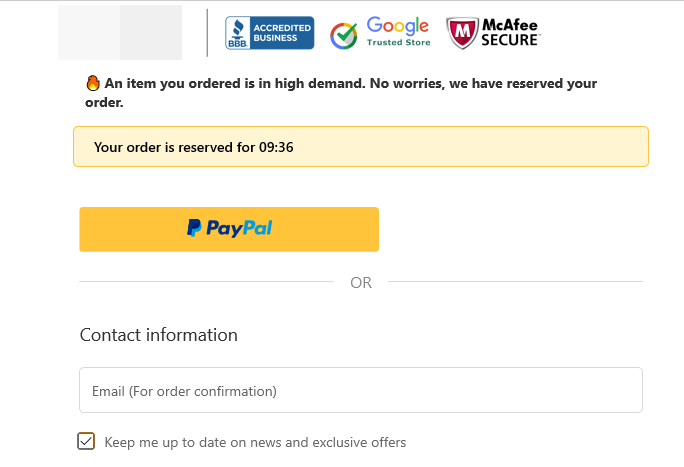In the background, the image features a white backdrop. In the top left corner, there are two squares side-by-side: one in darker gray and the other in lighter gray, separated by a thin gray line. Adjacent to this is the "Accredited Business" badge from the Better Business Bureau, displayed in blue and white.

Next to the BBB badge, you'll find the "Google Trusted Store" logo, a circle in red, yellow, green, and blue with a green check mark in the center. To its right, there's the "McAfee Secure" badge, featuring the iconic McAfee shield with a small fire symbol below it.

Beneath these logos, a message informs that "an item you ordered is in high demand" and reassures that "No worries, we have reserved your order." Below this message is a light yellow rectangle with black lettering that reads "Your order is reserved for 09:36."

Further down, there's a yellow button with "PayPal" written inside, in two shades of blue, dark and light. Underneath this button, a gray line separates the text "or," which sits flanked by two additional gray lines.

Below this, in black lettering against a white background, is the heading "Contact Information" in a light gray-blackish color. A long rectangle field labeled "Email (for your order confirmation)" follows. Lastly, there's a gray box with a black check mark in the center and text alongside it that reads "Keep me up to date on news and exclusive offers."